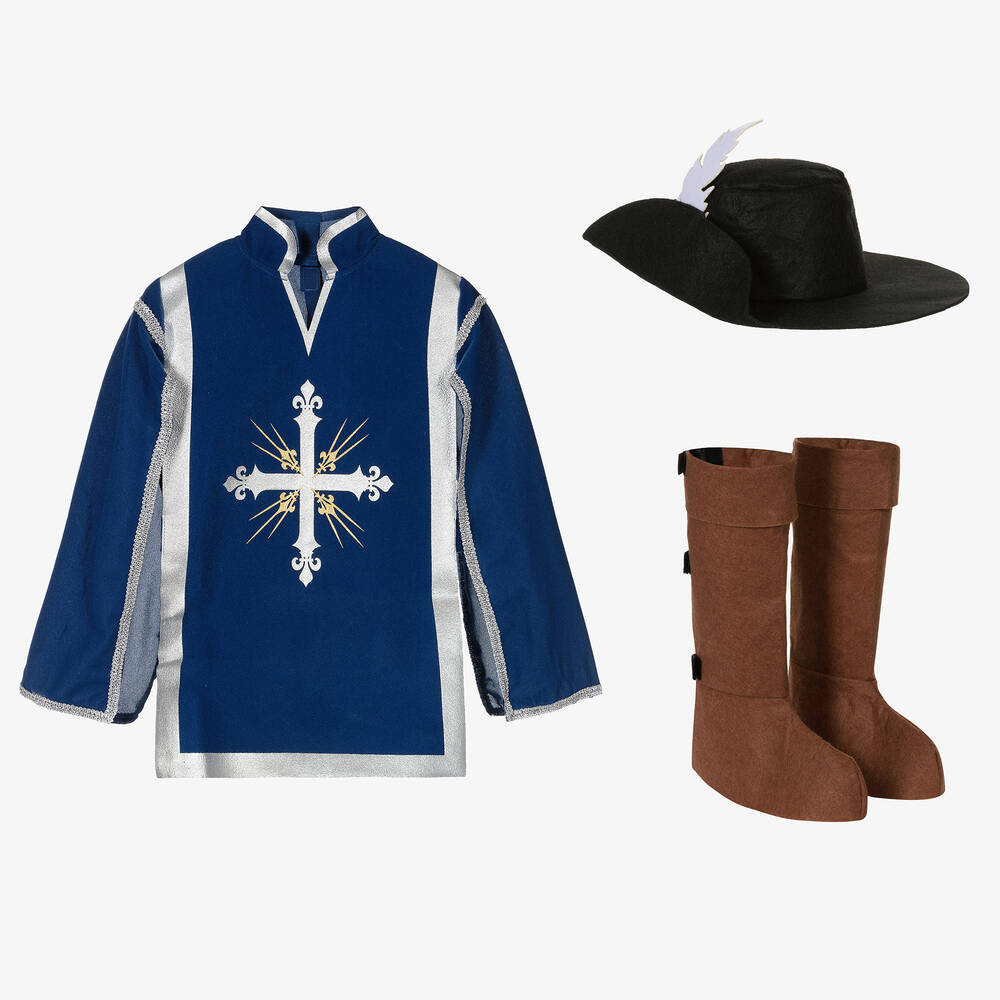In this image, set against a white background, there's an outfit comprised of various distinct items seemingly floating in space. On the left side, a dark blue, long-sleeve jersey with shiny, satin-like white trims, including a slight v-neck, captures attention. The jersey is adorned with a prominent white cross at the center, embellished with yellow lines radiating from behind in a pattern reminiscent of sparks. To the right of the jersey, a pair of knee-length, brown suede-like boots are displayed, notable for their smooth texture and unique design without a clearly defined sole. Above the boots, there is a black hat with a broad brim, featuring a striking white feather sticking out from the top. The boots, hat, and jersey are all meticulously detailed, highlighting the elaborate components of this intriguing outfit.